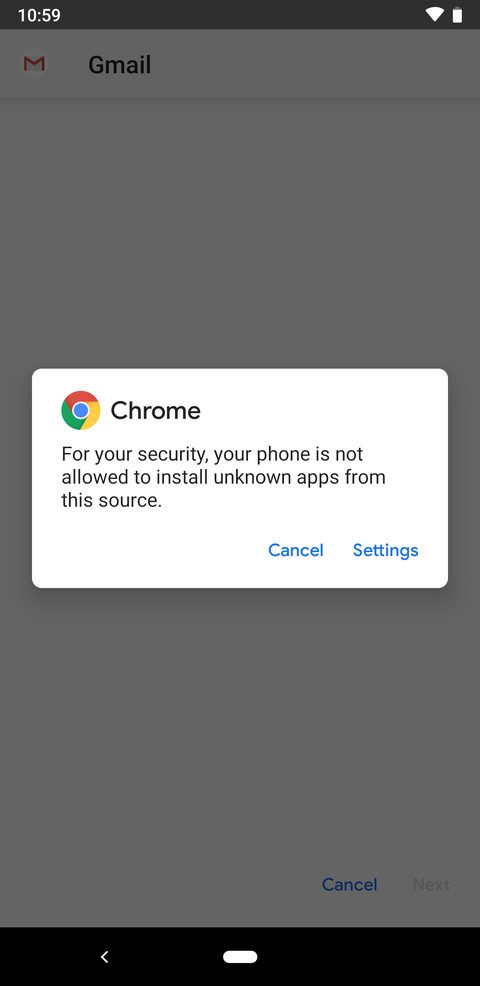The image is a detailed screenshot of a smartphone display. At the very top, the status bar is visible, featuring a battery indicator, a signal strength icon, and a timestamp—all displayed in white font on a black background. Beneath the status bar, the primary screen has a grayscale overlay, dimming its content, but the Gmail logo and the word "Gmail" are faintly visible in the background.

Dominating the center of the screen is a prominent white pop-up box related to the Google Chrome browser. In the top left corner of the box, the Chrome logo is clearly displayed next to the word "Chrome," highlighted in bold black text. The message within the pop-up reads: "For your security, your phone is not allowed to install unknown apps from this source." Below the message, there are two options presented—one to cancel the action and another to navigate to the settings to possibly allow the installation. The overall context indicates that the user attempted to install an app, but the smartphone's security settings are preventing the installation.